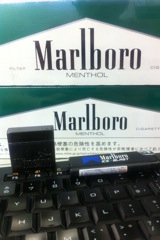The image shows two packs of Marlboro menthol cigarettes prominently displayed on a black keyboard with white letters. The cigarette packs feature a green top transitioning into darker green splotches, followed by a white band with the Marlboro logo in bold black letters and the word "menthol" underneath in light gray font. One pack is placed atop another, slightly obscuring the text. Adjacent to the cigarette packs, a blue magic marker and a pen rest on the keyboard. Visible keys on the keyboard include letters like 'U', 'Y', 'I', 'O', 'P', 'H', 'J', 'K', 'L', and a semicolon key. Additionally, a square-shaped device, which could be a type of camera, is also present near the cigarette packs. The scene suggests an indoor setting, potentially at a workstation with a connected laptop or desktop computer.